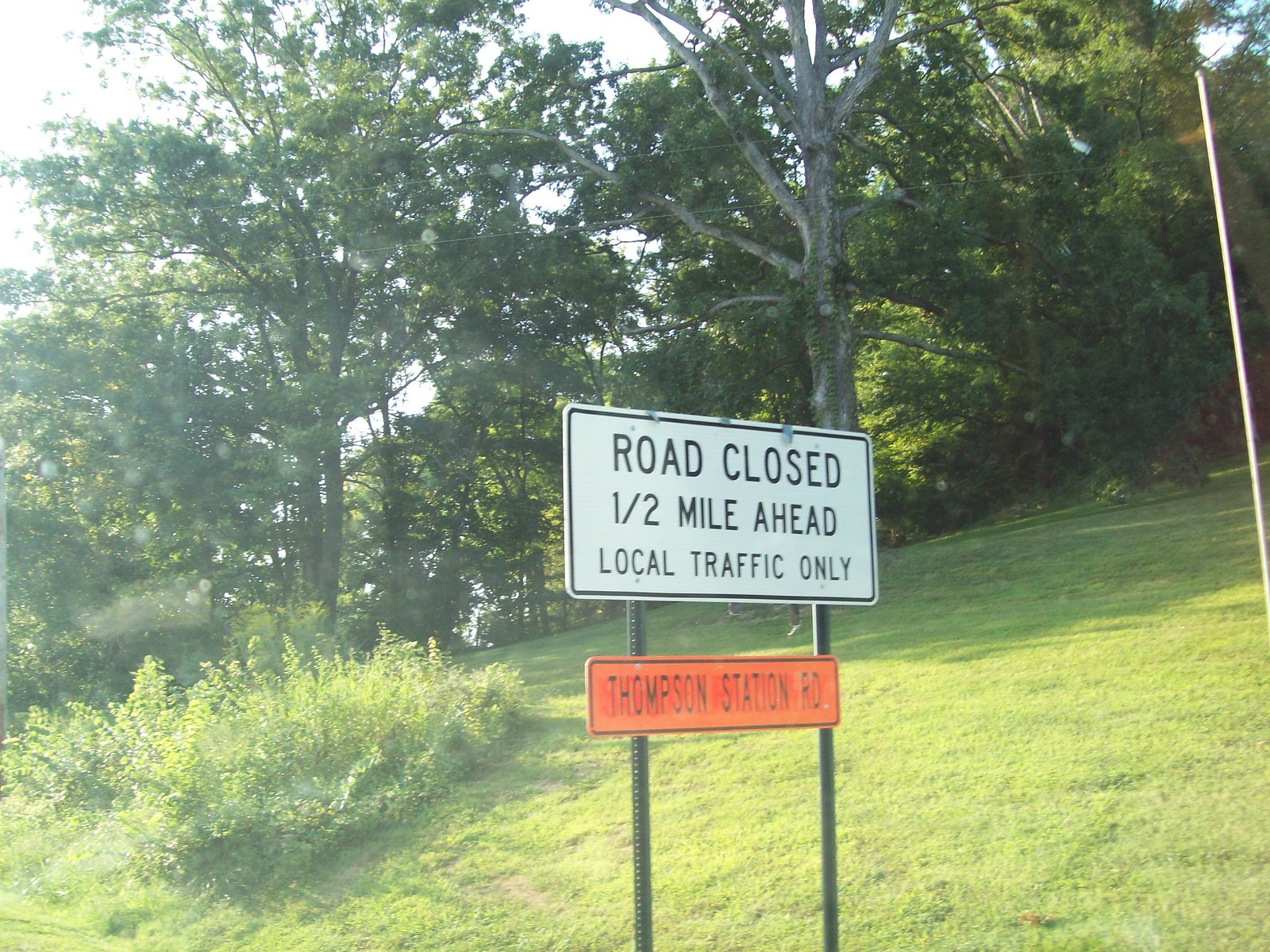A scenic green hill with meticulously maintained grass forms the centerpiece of the image. A large, lush bush stands prominently on the slope, accompanied by a group of towering, bushy trees that dominate the background. To the side, a silver pole rises conspicuously. The sky is a subdued light gray, with occasional glimmers of sunlight filtering through the clouds. In the foreground, a road sign with a green post and a white face bordered in black is visible, displaying the message "Road Closed One Half Mile Ahead, Local Traffic Only" in clear black letters. Further down, an orange sign bordered in black catches the eye, announcing "Thompson Station Road."